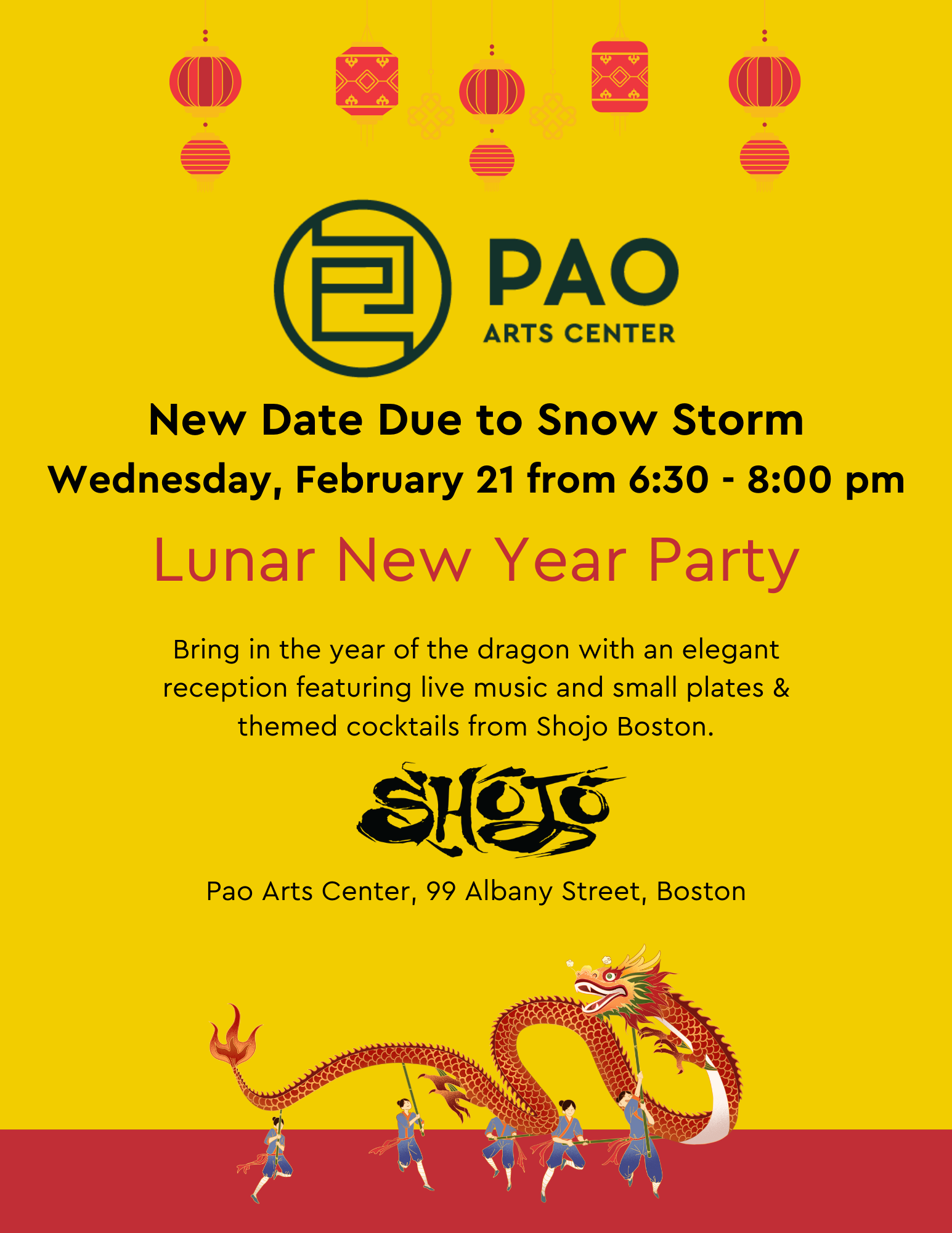This portrait-oriented event flyer for the POW Arts Center features a bright yellow background adorned with red Chinese lanterns at the top. The prominent header at the top displays "POW" in large, bold letters, with "Arts Center" in smaller font underneath, accompanied by a black circular logo with a geometric design to the left. Below this header, a notice in black font announces a new date due to a snowstorm: Wednesday, February 21st, from 6:30 to 8 p.m.

A striking red-font headline in the center reads "Lunar New Year Party." Following this, a paragraph invites guests to "bring in the Year of the Dragon with an elegant reception featuring live music, small plates, and themed cocktails from Shoujo Boston." The Shoujo logo, in a stylized paintbrush font, is positioned underneath the paragraph. At the very bottom, the flyer provides the address: "POW Arts Center, 99 Albany Street, Boston."

The lower section of the flyer features a dramatic large red dragon puppet, operated by five people dressed in blue, holding sticks that control its movement. This vignette is set against a red horizontal stripe at the bottom. Overall, the flyer skillfully combines vivid colors and detailed information to promote a festive celebration of the Lunar New Year.